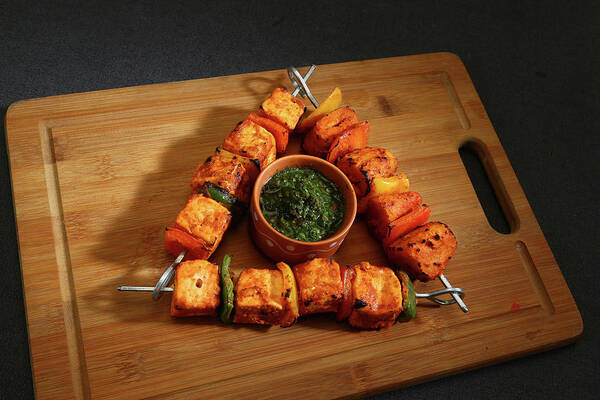The image captures a meticulously arranged culinary scene set against a dark, possibly black, backdrop. At the center is a wooden cutting board with an inset handle on the right side and a groove tracing its outer edge. Three metal skewers, featuring almost perfectly cubed pieces of meat—either pork or chicken—alternate with slices of vibrant green, yellow, and red bell peppers, forming a visually striking triangular display. The skewers, resembling traditional shish kebabs, intersect in a triangular formation. Positioned centrally within this triangle is a small, reddish-brown clay bowl containing a vividly green, pesto-like sauce made from fresh herbs and oil. The presentation, likely intended for social media or a food blog, showcases the food on a dark, contrasting surface, emphasizing the colorful and neatly arranged ingredients.